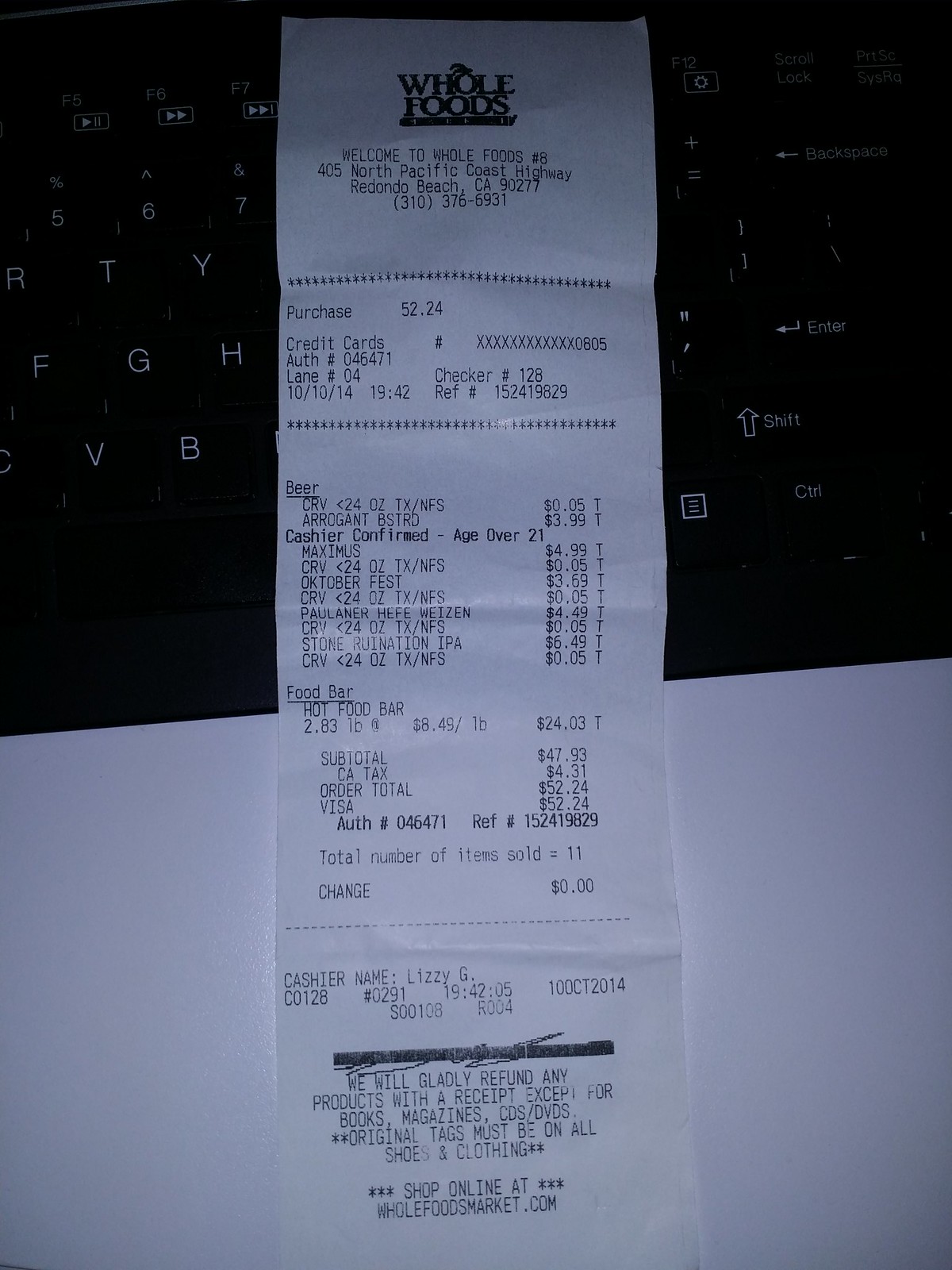A close-up photograph of a Whole Foods Market receipt from October 2014, captured in low light, resulting in a slightly blurry image. The receipt details a shopping experience at the Redondo Beach, California location. The total amount spent is $52.24, with 11 items listed. The top section welcomes customers to Whole Foods and provides the store's address. Several of the items appear to be priced at just a few dollars each, suggesting the purchase of various low-cost products, likely fruits or similar perishable goods. Notably, a significant portion of the total—nearly half—is attributed to purchases from the store's food bar, amounting to almost three pounds of prepared food.